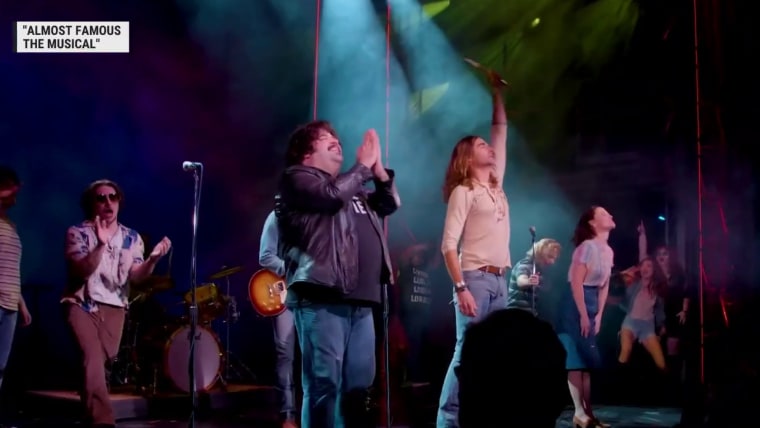Under the dim spotlights, a celebration unfolds on stage against the backdrop of the Almost Famous the Musical title in the upper left corner of the photograph. The central figures, highlighted by the lighting, include a hefty man in a black leather jacket, black undershirt, and light blue jeans, alongside a long-haired man in a beige top, brown belt, and light blue jeans, enthusiastically holding up what resembles a wooden spoon. To their left, a man sporting brown sunglasses and a brown hair claps his hands next to a microphone stand, while to their right, a woman with a long blue skirt and tucked-in white shirt takes a bow. In the backdrop, partially obscured by dim lighting, musicians including a guitarist and a drum set can be spotted, with additional figures extending their arms, creating an energetic post-performance atmosphere.